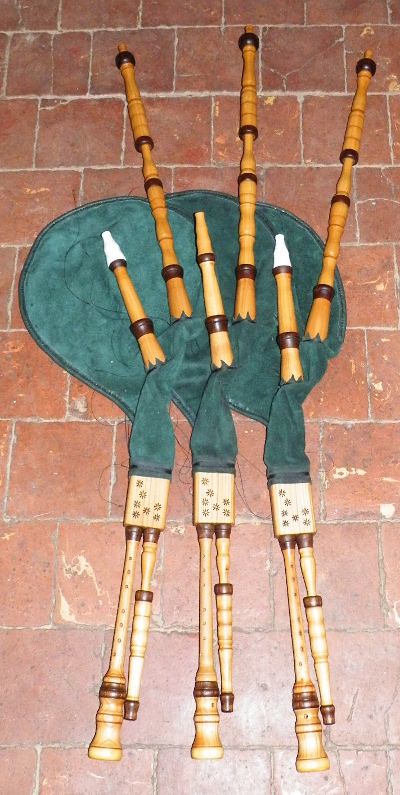This is a detailed photograph of three bagpipes laying flat on a red, square, brick-tile floor. The green velvet bags of the bagpipes range from light to dark green, giving a rich textural appearance. At the top of the image, the wooden pipes, which are in a variety of brown shades, are layered over each other. Some pipes have darker rings near the mouthpieces, adding a touch of distinction. The bottom section features additional pipes with lighter shades of brown and small floral decorations, adding to the intricate visual. The photograph appears to be taken from above, showing the intricate arrangement and fine details of this traditional Scottish instrument. The older-looking floor surface with its aged brick layout provides a contrasting backdrop to the vibrant details of the bagpipes.